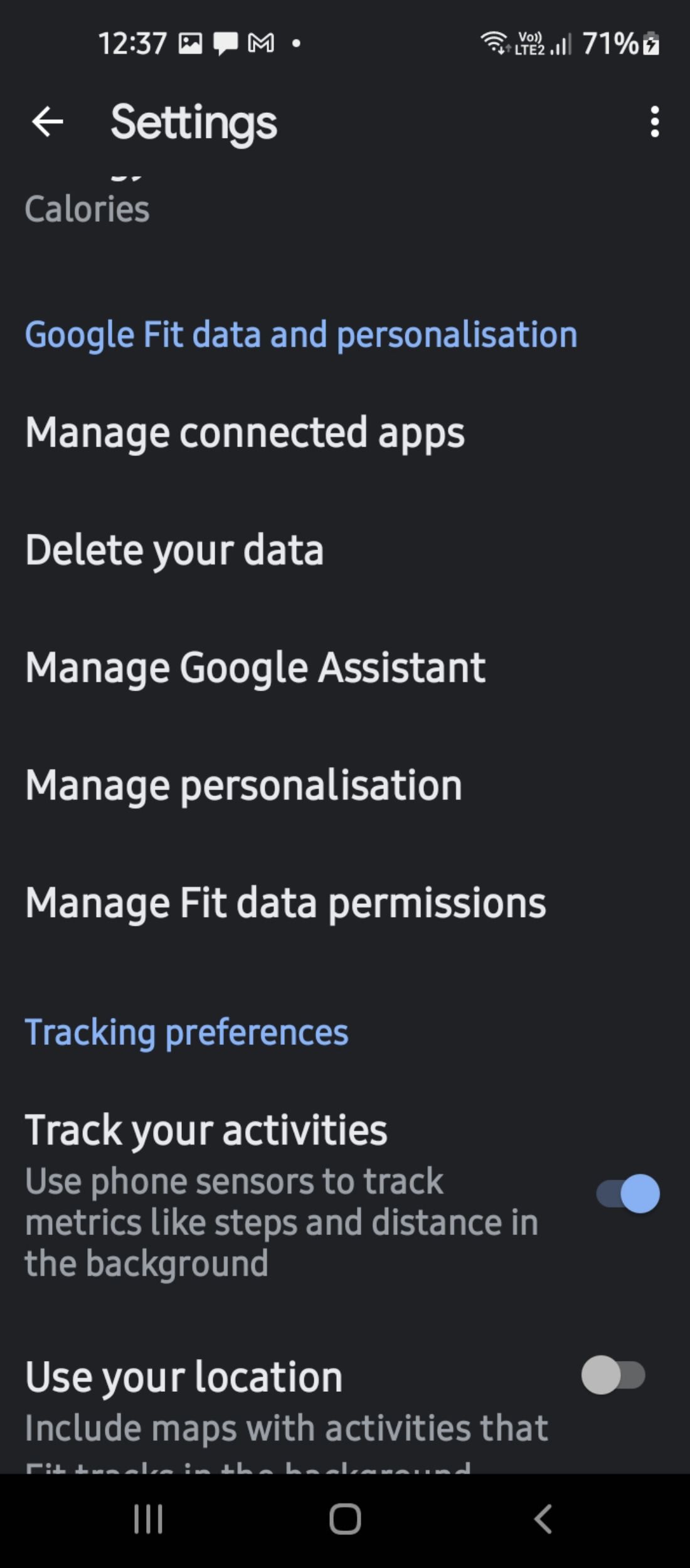Screenshot of a smartphone at 12:37 PM displaying a settings menu with various icons and status indicators. The top bar includes icons for cellular signal (with 3 bars filled), a partially filled battery at 71%, and Wi-Fi with a filled downward arrow and an empty upward arrow, indicating traffic status. 

Below the status bar, the screen shows "Settings" with a left-facing arrow and a three-dot menu icon on the far right. 

The menu options listed in blue and white text include:
- "Calories"
- "Google Fit data and personalization"
- "Manage connected apps"
- "Delete your data"
- "Manage Google Assistant"
- "Manage personalization"
- "Manage Fit data permission"

In blue text, it says "Tracking preferences," followed by "Track your activities" in white. Below, in gray text, is the description "Use phone sensors to track metrics like steps and distance in the background," with the toggle switched on.

Following this is "Use your location" and "Include map with activities" (the latter cut off and illegible), with the setting turned off.

At the bottom, the generic Android navigation bar includes icons for a three-line menu on the left, a square tab in the center, and a back arrow on the right.